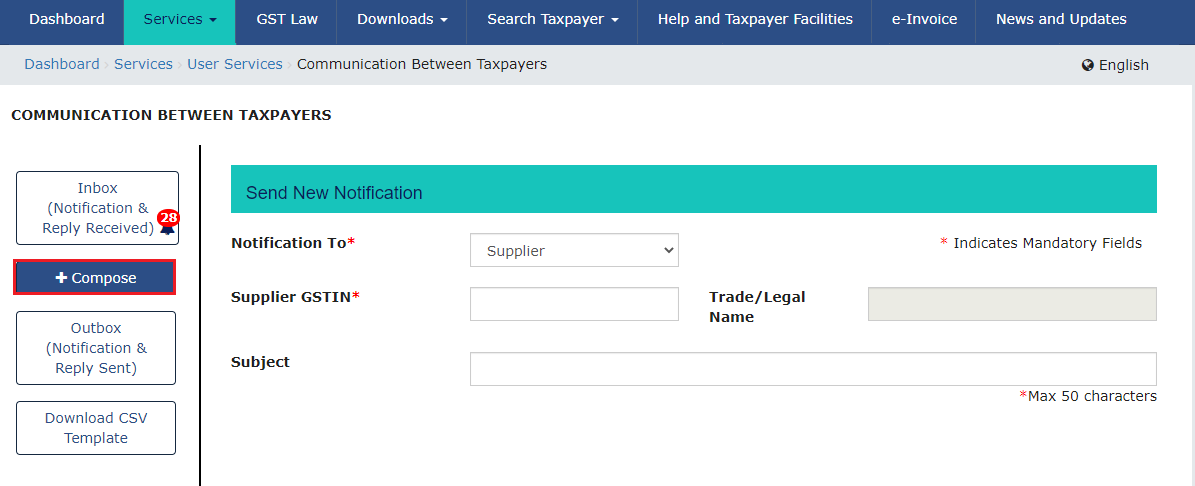This image is a detailed screenshot of an account dashboard page on a website, likely related to GST (Goods and Services Tax) management. At the very top, the header features a navy blue background with the menu items written in white. 

- On the left side of the header, the text "Dashboard" is displayed in white.
- Next to it, a blue rectangle with aquamarine tones displays "Access Services" in blue font, accompanied by an inverted triangle indicating a drop-down menu.
- Following this, the background returns to navy blue with the menu items "GST Law," "Downloads," "Search Taxpayer," and "Help," each paired with an inverted triangle for additional options.
- A section marked "e-Way Bill System" is present without a drop-down menu.
- On the right side of the header, there's a prompt labeled "New Return Trial" with another drop-down menu.

Below the header is a gray strip containing more options:
- From left to right: "Dashboard," "Services," "User Services," and "Communication Between Taxpayers."
- On the far right, there's an option for "English," indicated by a globe icon.

The main body of the page has a white background. On the left side, in black capital letters, the text "Communication Between Taxpayers" is displayed. Below this, a side bar includes the following menu items outlined in gray:
- "Inbox" with a notification bell icon, displaying a red circle with the number 28, indicating 28 new notifications.
- A blue rectangle that says "Compose," outlined in red.
- Additional options: "Outbox," "Notification," "Reply Sent," and "Download CSV Template."

In the center of the page, there is a header in aquamarine green that reads "Send New Notification." Below this header is a blank form with fields for "Notification to the Supplier," "GSTN," "Trade Legal Name," and "Subject."